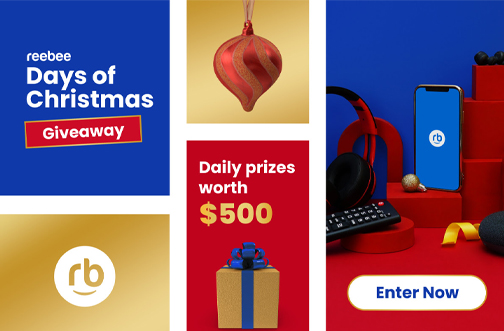This image is a promotional screenshot from a website advertising a Christmas sale for consumer electronics, featuring a series of festive ad boxes:

1. The first box has a blue background and reads "Reebee Days of Christmas." A red banner overlay says "Giveaway."
2. Below it, a box with a gold background displays the Rebee logo (R-E-B in a white circle with a smile line beneath it). A red ornament shaped like an inverted teardrop with a white background is centered at the top.
3. The next box has a red background and announces, "Daily Prizes Worth $500." A graphic of a gold gift box with a blue bow complements the text.
4. The final ad banner, situated to the right, features a blue background with various electronics: a phone displaying "R-B", a black and red headset, a remote control, and several red gift boxes atop red platforms on a red countertop. An "Enter Now" button in white is positioned at the bottom.

Overall, the image effectively communicates various elements of a Christmas sale event hosted by Reebee, highlighting daily prize opportunities and tech giveaways.